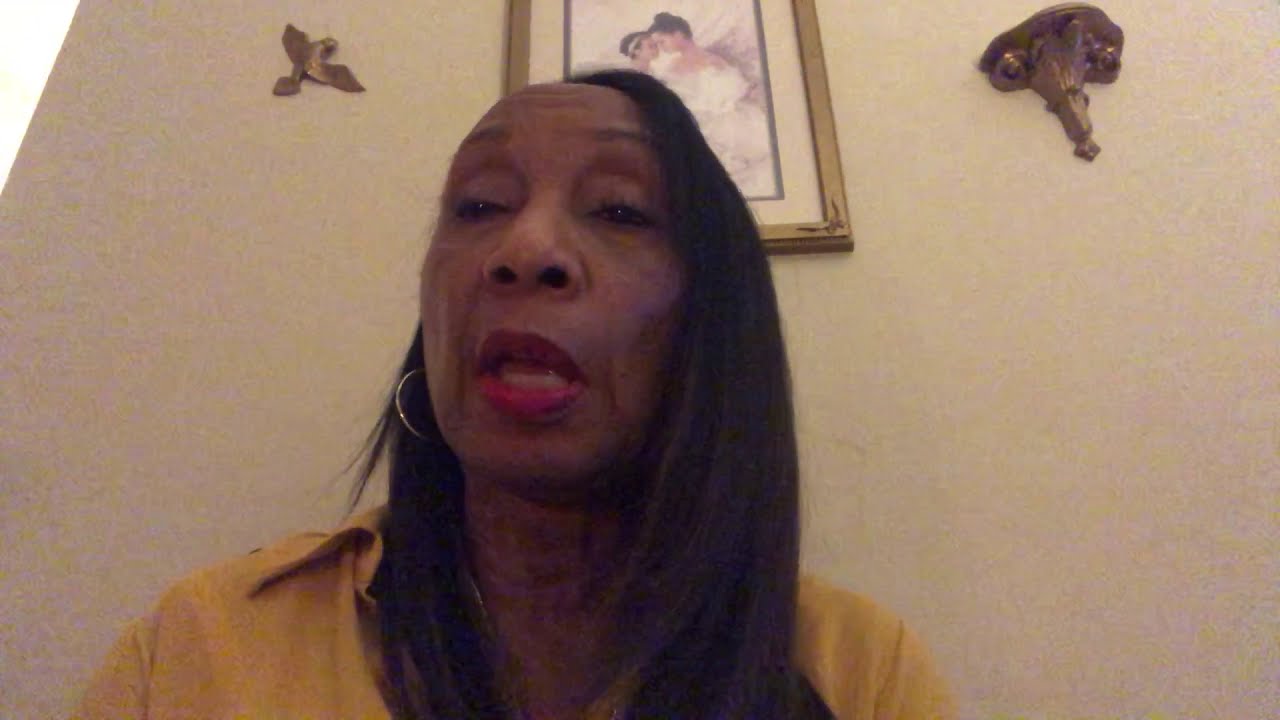The image appears to be a still from a low-quality, grainy video, possibly taken in low light or with a poor webcam, adding a significant amount of digital noise to the scene. The focus is on an older African American woman with long black hair that cascades down past her shoulders. On her right side, the hair drapes fully, while on the left side it is partially tucked behind her ear. She is wearing a large silver hoop earring on the visible ear, and her attire consists of a yellow collared blouse that features a thin chain necklace. Her face is adorned with thin black eyebrows and very pink or red lipstick. The background reveals a taupe or beige-colored wall. Mounted on the wall behind her is a framed photograph of a woman and a child, encased in a gold frame. To the left of the photograph is a golden bird decoration, and to the right, a small golden or bronze curio shelf, which appears to be empty. The woman's posture is slightly tilted back, giving a view into her nostrils, as she looks and speaks toward the camera.